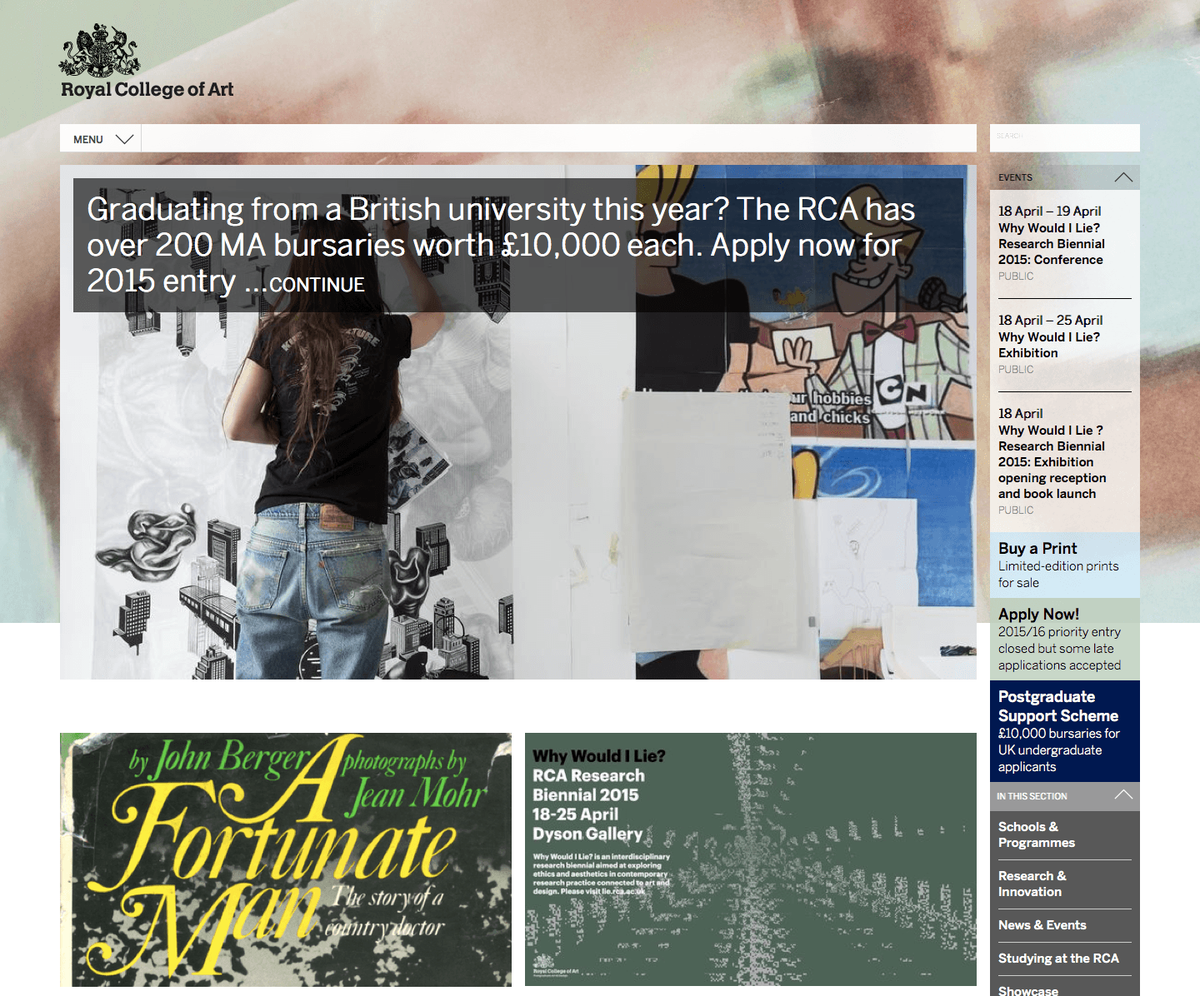The image showcases the Royal College of Art website. In the upper left-hand corner, the "Royal College of Art" logo is prominently displayed. The top section of the image features a blurred background dominated by skin tones, though it's hard to discern specific details. 

Directly beneath the Royal College of Art banner is a white bar. Positioned on the left side of this bar is a menu icon accompanied by a dropdown arrow. Adjacent to it is a vertical events calendar, which presents various upcoming events through a series of date blocks.

The main content area to the right of this white bar is divided into three sections. The most prominent section at the top is labeled "Graduating from British University this year?" It contains information about the RCA offering more than 200 MA bursaries, each valued at £10,000, for the 2015 academic entry, urging viewers to apply now.